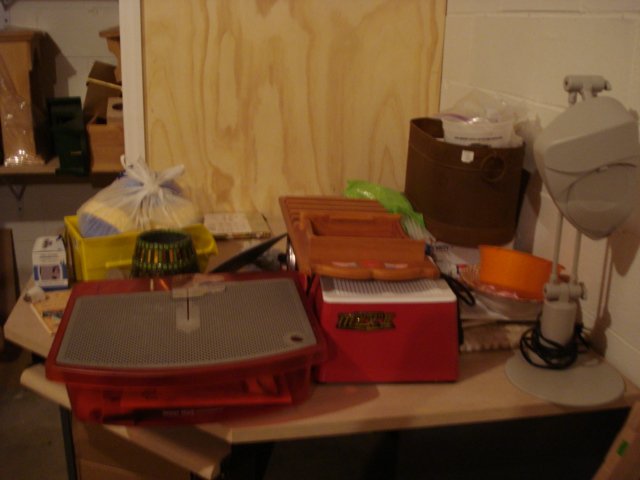The photograph portrays a corner of a room with light ivory cinder block walls. Against these walls, a corner-style desk with a light tan top and a dark brown base is situated. This desk features a central drawer. 

On the adjacent wall behind the desk, there's a piece of plywood in a blonde hue. The desk itself holds a varied assortment of items piled in a seemingly haphazard manner. Notably, there is a clear orange plastic container with a gray inset in its lid, housing slender books. Beside it, a brown plastic bucket contains several items, including a yellow plastic cube. Additionally, a white grocery-style plastic bag, tied at the top, is present. 

A tan-colored lamp with an adjustable arm and a black cord coiled around its base stands on the desk. Strewn about are more items: another orange plastic container, a red square box with a white lid, and various other plastic objects and papers stacked together in an unorganized fashion.